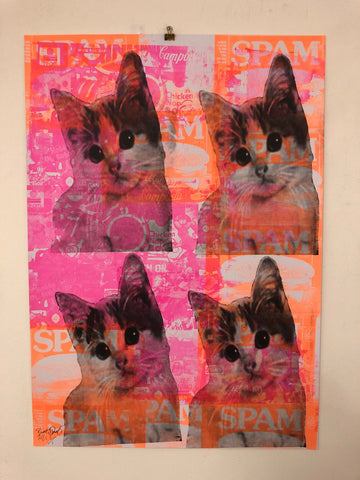The vertically aligned rectangular image showcases a detailed and colorful collage hung on a light brown wall, secured by a single binder clip attached to a nail. The centerpiece of this artwork is a poster divided into four symmetrical sections, each featuring the identical image of an adorable black and white cat with a white face and underside, positioned centrally within the composition. Each cat image is set against a differently colored background, exclusively using shades of pink, orange, and white, providing a vibrant and playful contrast.

Above the collage, just beneath the clip, the word "Campbell's" can be seen, hinting at a possible theme related to food products. Amidst the collage, the text "spam" repeatedly appears in various colors, further emphasizing this theme. The arrangement is framed with a light gray border, adding a subtle yet defining outline to the piece. Each of the four sections presents the cat with its head tilted, long whiskers accentuated, and a direct gaze towards the viewer, creating a cohesive and engaging visual narrative.